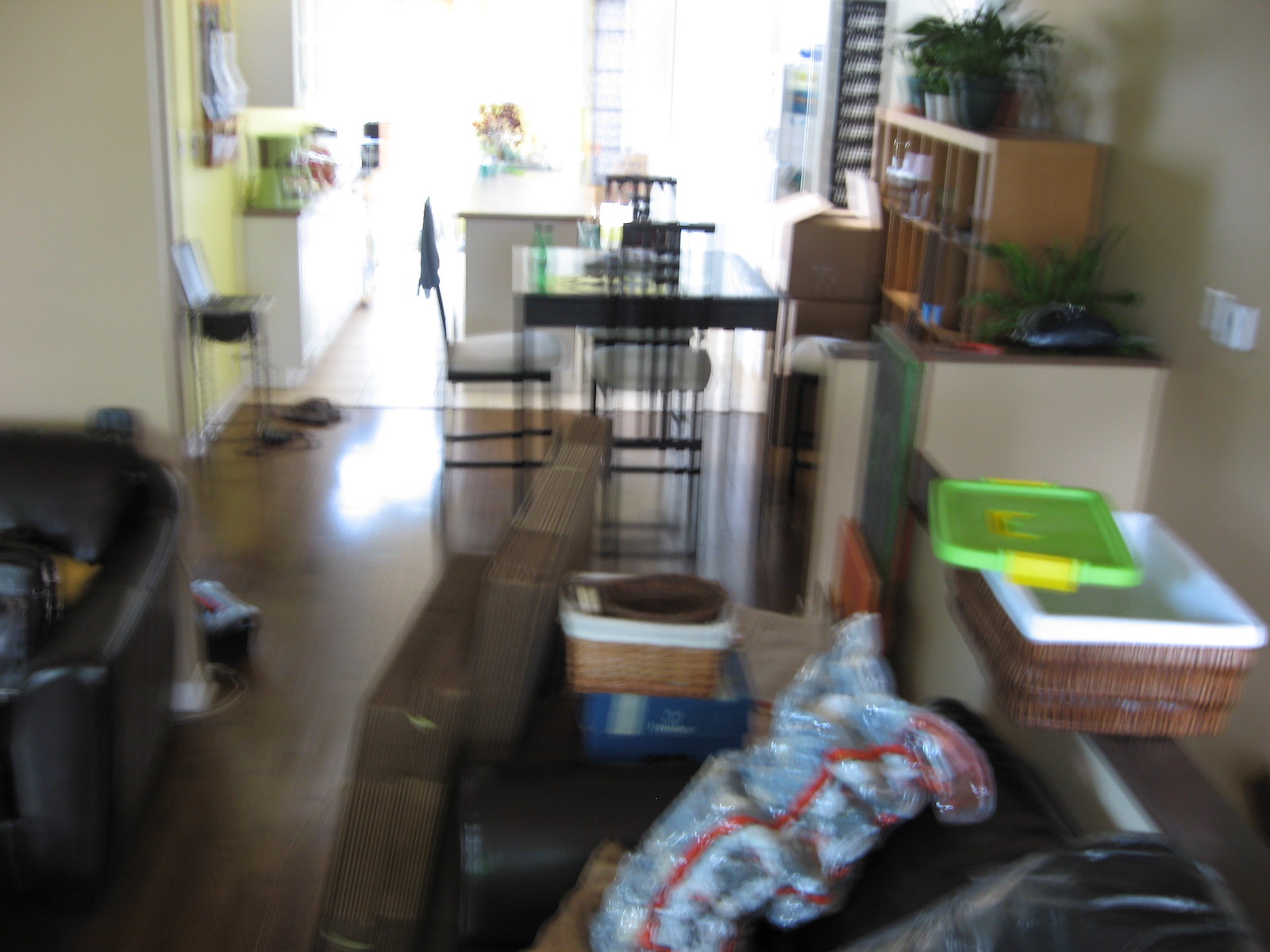This image captures a somewhat cluttered and blurry view of an apartment, detailed as follows: The living area features two black couches positioned against a tan wall, above which a small shelf is installed, creating a nook-like effect. A wicker basket is perched on a room divider wall near the couch. The dining area, centrally located in the open-plan kitchen, includes a table with a trio of tall chairs. A child's high chair resides against the kitchen wall. On the right side of the room, a bookshelf adorned with plants occupies the wall space, accompanied by an office-style set of file drawers, also topped with plants. 

Partially visible, the kitchen showcases a predominantly white decor with an island and a light green mixer standing out on the countertop. A green bottle, possibly a Sprite, alongside various unidentified items, clutter the dining table. Resting on one of the couches is a bag containing a knitted Afghan blanket, exhibiting patterns in light blue, red, and white. Discarded or yet-to-be-unpacked boxes, potentially indicating a move, are stacked between the kitchen and living room along with another wicker basket filled with miscellaneous objects. Next to the half-wall separating the kitchen from the living room lies a small basket.

Additional features include a wooden floor throughout the apartment and a thermostat located on the right-hand side wall. The overall impression suggests a lived-in, slightly disorganized space perhaps in the midst of a transition.